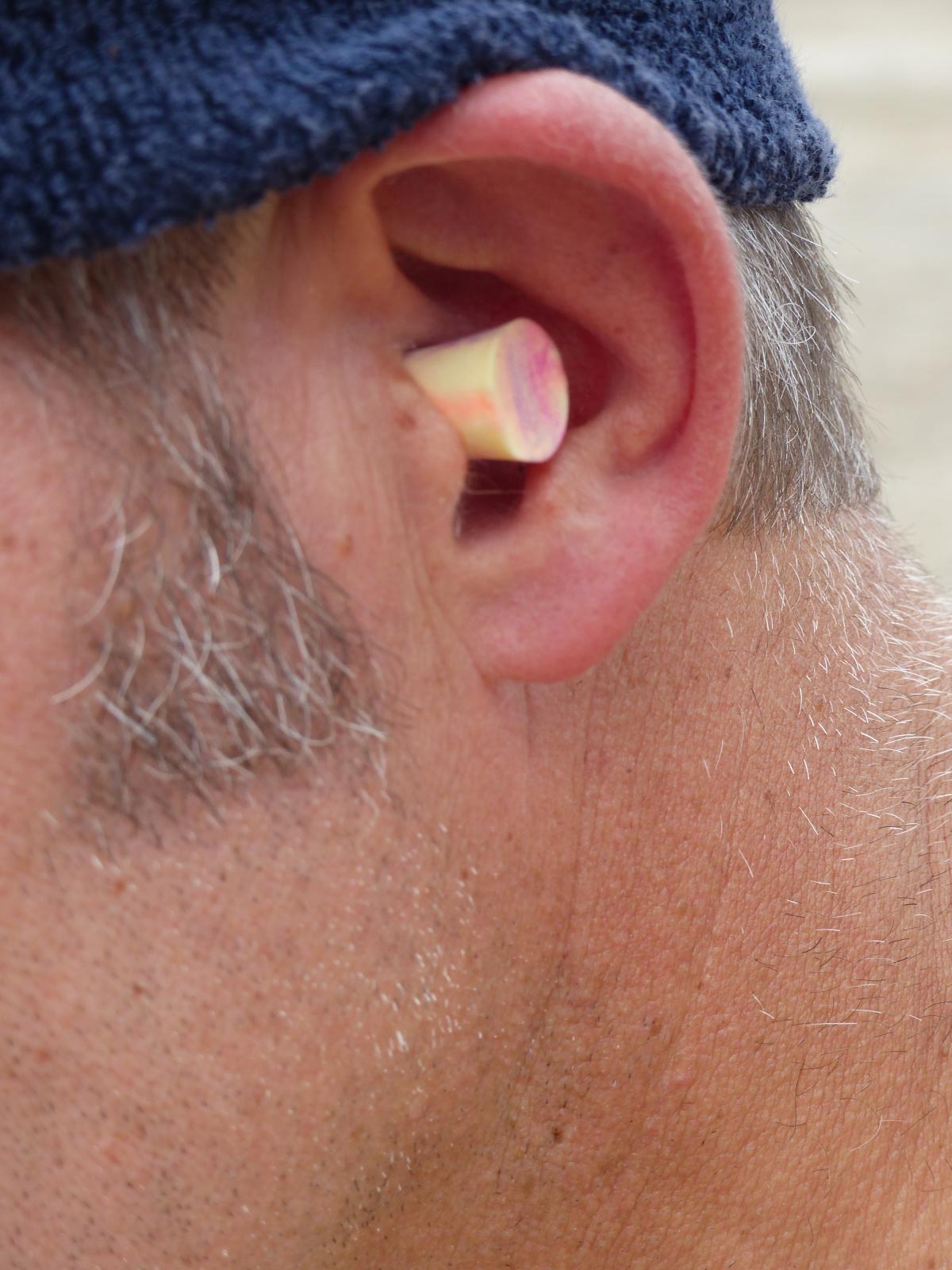This is an incredibly detailed close-up photograph of an older Caucasian man wearing a foam earplug. The image primarily focuses on the left side of his head, capturing everything from above his ear down to his neck. He is donning a navy blue knit cap, which sits snugly on his head, shrouding the top of his ear. His short hair is a mix of silver and white shades, with darker gray sideburns extending down to the length of his ear. His ear appears notably red, suggesting it might be cold. The light yellow earplug in his ear displays hints of purple and pink at the tip. The skin on his neck and the back of his head, with visible texture and slight stubble, points to an imminent need for a shave. Despite the proximity of the shot, the ear and earplug are slightly out of focus, while the main clarity rests on his neck and the silver strands of his hair.